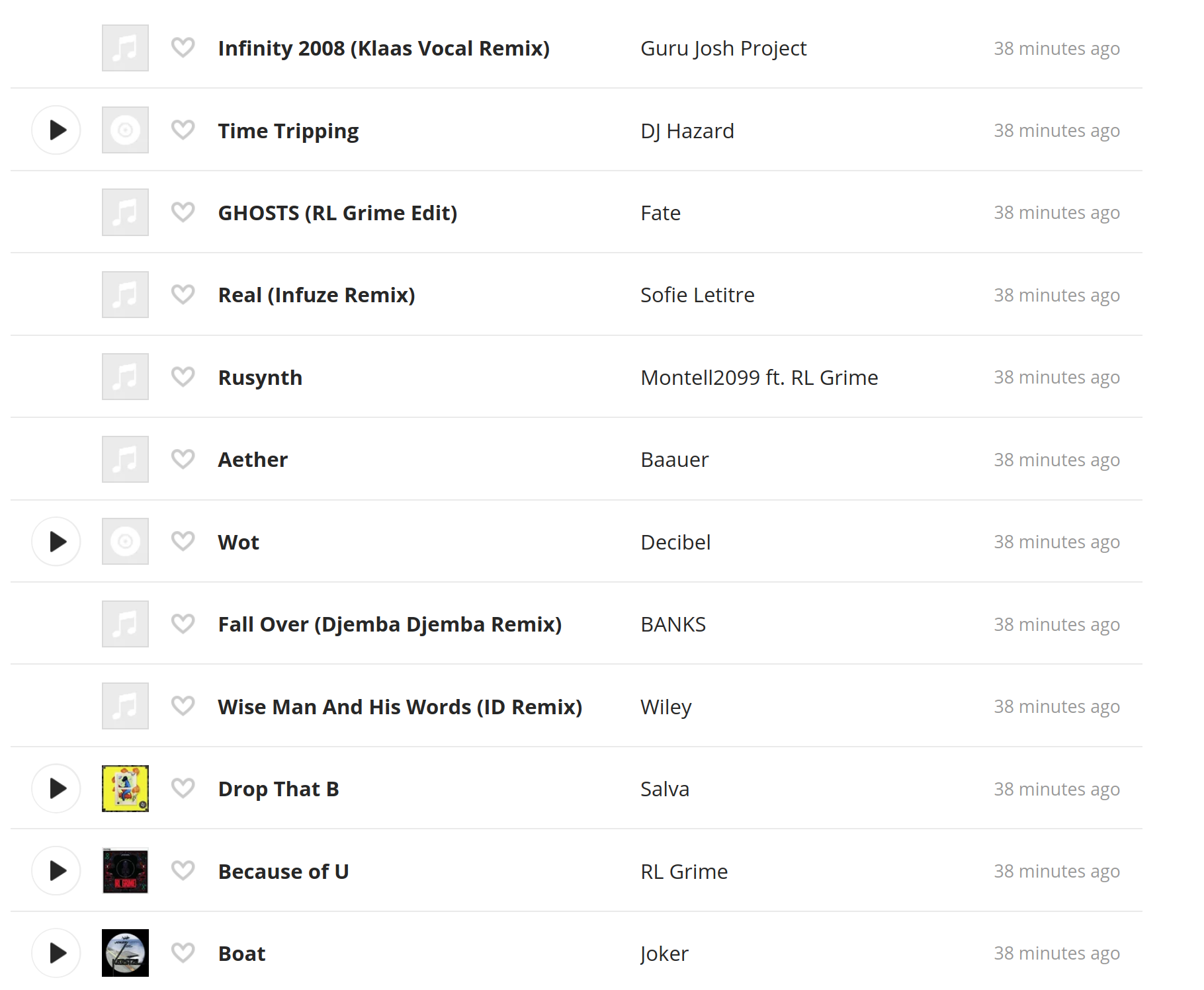This image features an artistic depiction of a playlist or music compilation with several tracks listed. At the top of the list is "Infinity 2008 (Class Vocal Remix)." Following this, the title "Time Tripping Ghost (RL Grime Edits)" is displayed. Then you see "Real Infused Remix" attributed to Russ Bruce Smith. The compilation continues with "8th Year," followed by "What Follows Her (DJ Amba Remix)." Next, "Wise Man and His Words (ID Remix)" appears, succeeded by "Drop That." The list concludes with "Because of You" and "Boat." The tracks are presented in a curated order, each with its specific remix or edit identifier, suggesting a diverse and modern musical selection.